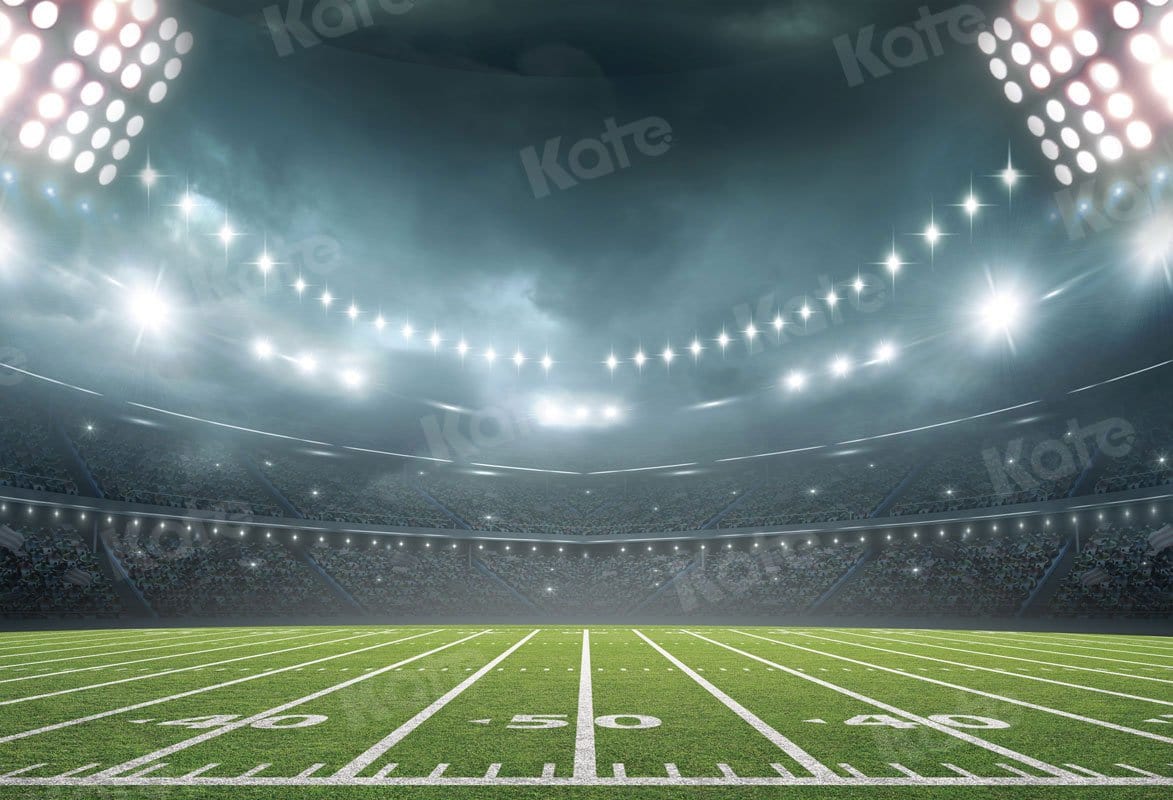The image showcases a vibrant, nighttime scene of a football stadium captured at the 50-yard line. The green, grassy field is marked with prominent white yard lines, including the 40, 50, and 40 yards. Above, the black night sky sets a dramatic backdrop, while an array of bright white lights illuminates the entire stadium. These lights are positioned along the top edges of the stands and extend from large fixtures in the upper left and right corners. The stands appear filled with spectators, contributing to the energetic atmosphere, although one description suggests the seats might be empty. Adding a touch of artistic flair, a hazy effect with smoke engulfs the top of the stadium. Dominating the image is a watermark with the text "Kate" written across it.